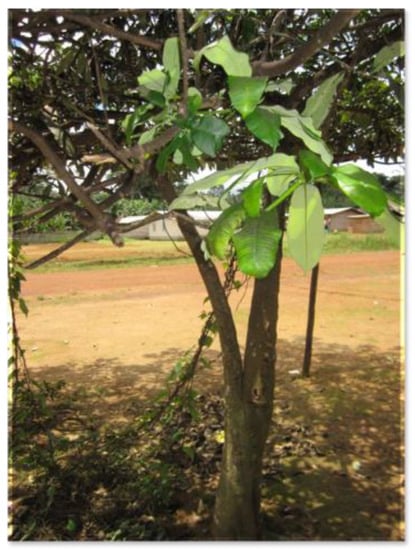In this outdoor scene, the foreground is dominated by a medium-sized tree, its trunk extending upwards and splitting into numerous branches adorned with leaves. The tree is flanked by vine-like plants, distinguishable by their very long, oval-shaped, and brighter green leaves, which contrast with the darker leaves of the tree itself. Light filters through the foliage, casting intricate shadows on the mostly dirt-covered ground and creating a sense of a sunny day.

Horizontally bisecting the image is a dirt road, beyond which lies a grassy area. Further back, partially veiled by the tree's thick cover, is a white building that could be a house, barn, or farmhouse—its exact shape remains obscured by the dense leaves. The background culminates in a line of distant trees, adding depth to the tranquil rural setting. No cars or people are visible, emphasizing the serene, uninhabited atmosphere captured in the photograph.